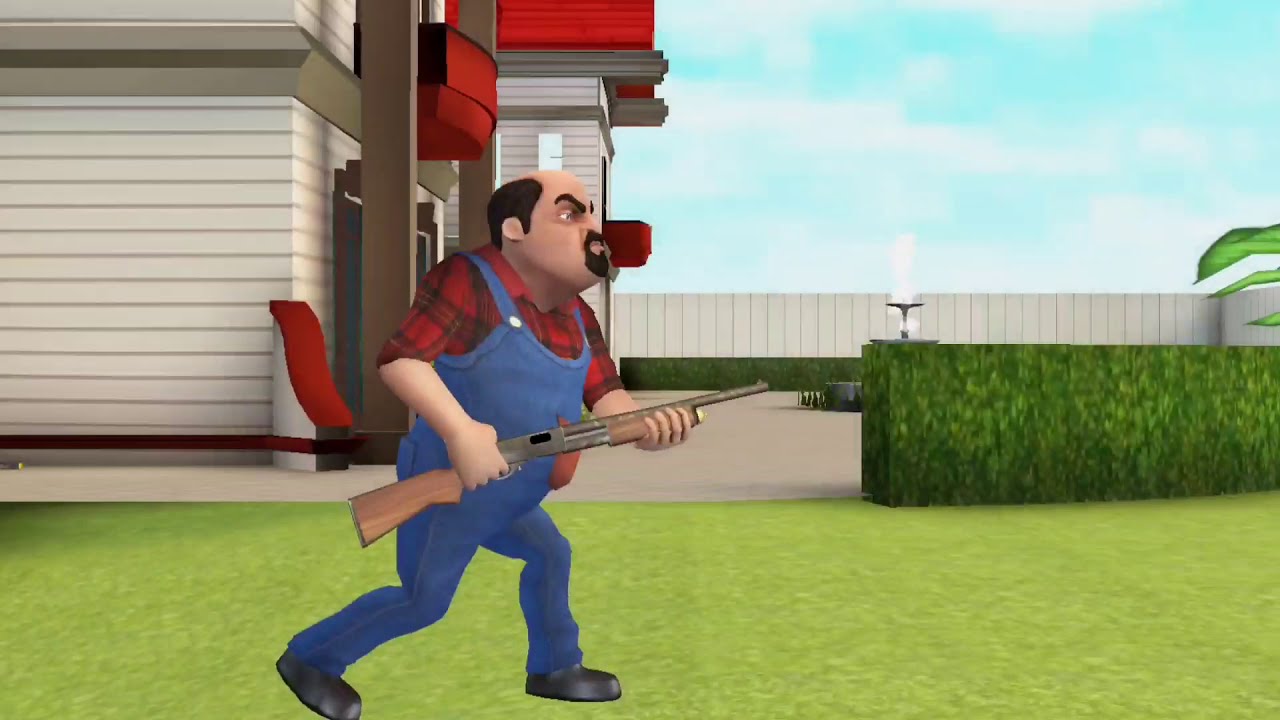The image is a computer-generated 3D cartoon screenshot from a video game, depicting a heavyset, partly bald man with black hair, a goatee, and dark eyebrows. He wears a long-sleeved red and black checkered flannel shirt with blue denim overalls or suspenders. The man, who has an angry expression and is furrowing his eyebrows, is marching towards the right side of the frame while holding a shotgun with a gray metal bar and a brown handle. He stands on a perfectly flat, bright green lawn, with a green hedge marking the edge. In the background, a white, two-story house with beige trim, red awnings, and an upstairs deck with red siding is visible. Further beyond the hedge, there's a three-tiered fountain with water flowing and a white fence surrounding the backyard. The sky is blue with white clouds, and some leaves of a fern are also part of the background scene.